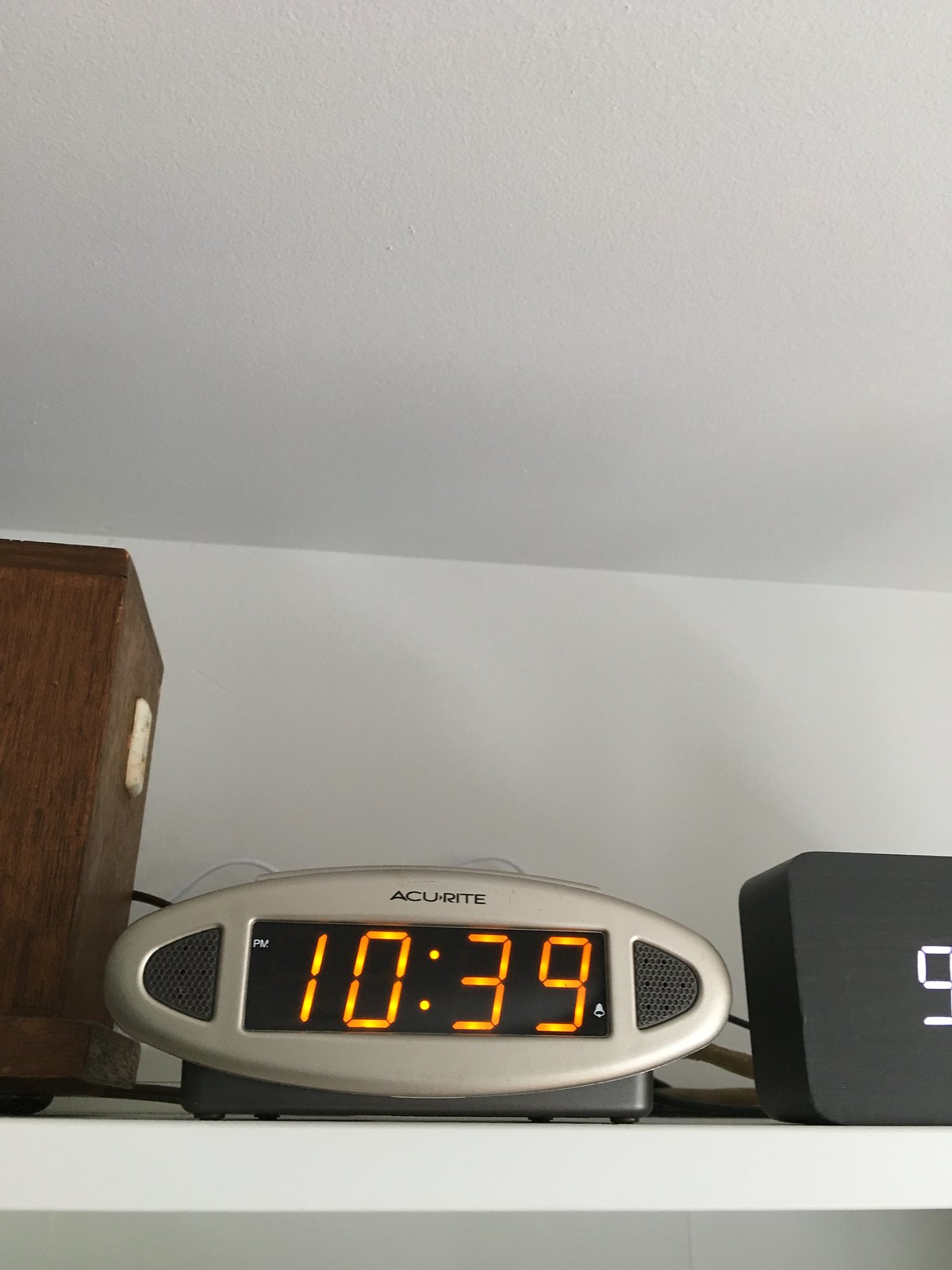In this rectangular photograph, the focal point is a beige-colored, oval-shaped LED clock situated on a white shelf mounted to a white wall. The shelf occupies the bottom section of the image. The wall meets the ceiling towards the center of the image, where the ceiling has a slightly bumpy texture and is painted the same white color as the wall. 

The LED clock, prominently placed in the center of the shelf, features black grates on its left and right sides, likely serving as speakers. The clock's central portion showcases a black rectangular LED screen displaying the time "10:39" in bright orange digital numbers. Above the screen, the brand name "ACCUWRITE" is boldly printed in all capital letters.

To the right of the clock, there is a small black rectangle with a white digital number "5". On the left side, there is a glimpse of a rectangular wooden brown box, partly out of the frame, adding a touch of warmth to the otherwise monochromatic setting. This detailed composition captures the simplicity and functionality of the space.